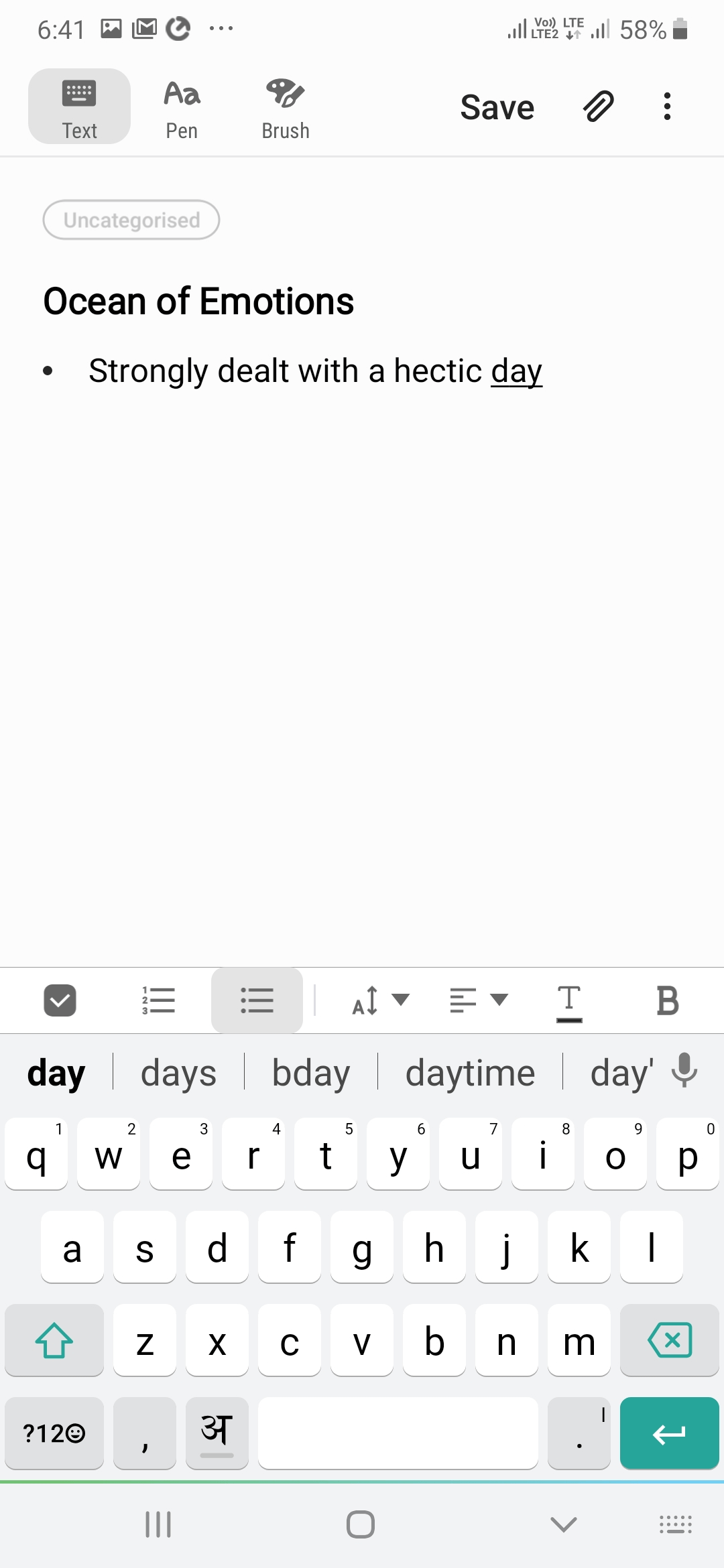The image displays a smartphone screen at 6:41 PM with a variety of UI elements. At the top of the screen, there are icons for a photo, cell signal bars, and a battery indicator showing 58% battery remaining. Below these indicators, various buttons are aligned horizontally, including a text button, a PEN button, a brush button, a save button, a paperclip icon, and a three-dot menu.

The screen displays the text heading “Uncategorized” followed by the phrase “Ocean of Emotions”. A bullet point is listed underneath, with the text “Strongly dealt with a hectic day,” where the word "day" is underlined. 

At the bottom of the screen, there is a virtual keyboard featuring white keys with black letters. Notably, the return key has a green arrow on it, while the backspace key has a green arrow with an X. There’s also a key with a left-pointing white arrow and several gray arrow keys. Below the keyboard, there is a green line followed by three vertically stacked lines, a circle icon, and a downward arrow. In the bottom right corner of the keyboard, there is an icon representing the keyboard itself. The underlined word “day” corresponds with the text prediction feature, suggesting terms for the user to select.

Overall, the image offers a detailed view of a smartphone interface in use, showcasing both functional icons and an example of text editing on the device.